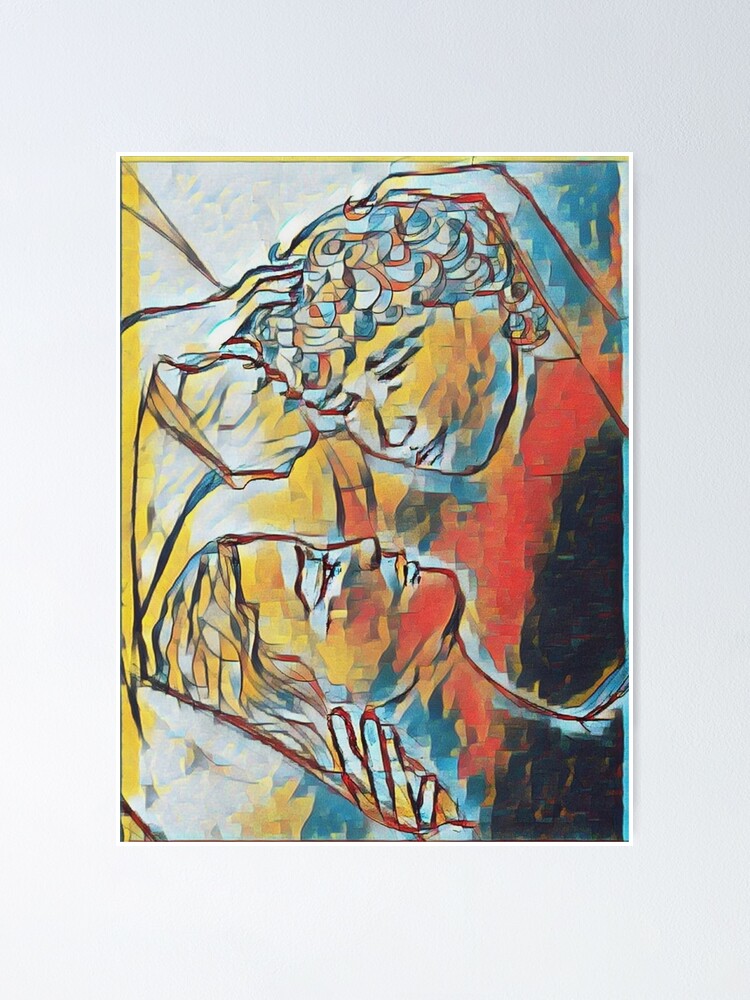This detailed painting, framed in a thin white or possibly gold frame, hangs on a light blue or gray wall. The artwork vividly captures a man and a woman in a tender, intimate embrace. The man, dressed in a red shirt, cradles the woman's neck as they gaze into each other's eyes with playful smiles, suggesting a forthcoming kiss. The painting's creative use of color transitions from dark shades on the right to brighter hues on the left, creating an intriguing layering effect. These colors—black, red, blue, tan, orange, yellow—render the figures in abstract tones, rather than their natural flesh colors. The nuanced depiction of their curly hair and the tender interaction, with the woman seemingly lying down and both playing with each other's hair, evokes a deep sense of closeness and contentment between the two.